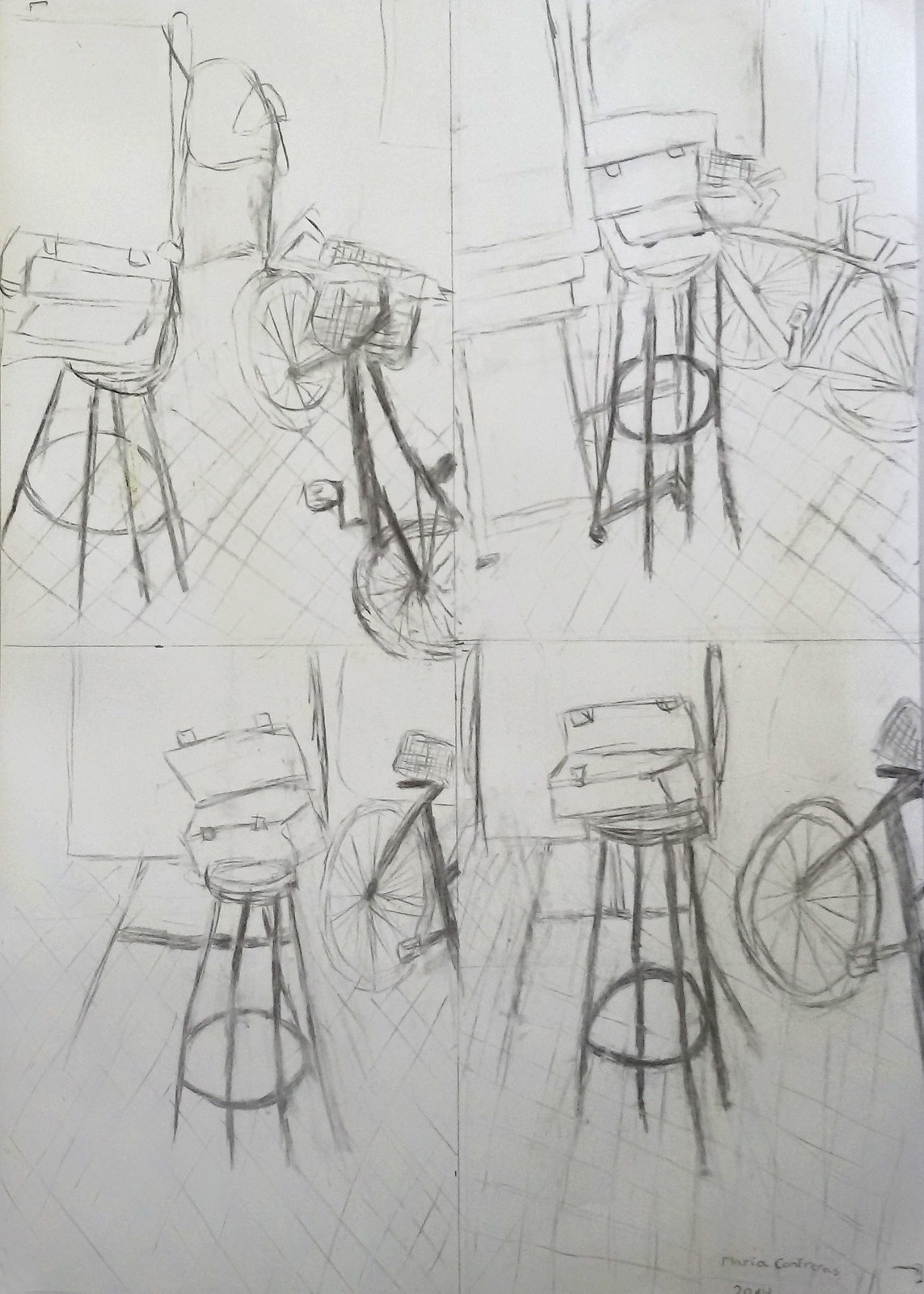This image presents a quartet of detailed pencil sketches, each capturing variations of a still life scene set within a simplistic, uncolored interior. The focal elements include a bar stool, an open toolbox, and a bicycle, all situated on a floor adorned with a diamond pattern. The sketches are arranged in a 2x2 grid, each offering a unique perspective of the same setting. In the upper left drawing, the bicycle occupies the lower left side. The upper right sketch shifts the bike further to the right, laying horizontally near the center-right. The lower left illustration portrays only the rear portion of the bicycle, positioned centrally. Similarly, the lower right sketch mirrors this view, focusing on the rear of the bike. Throughout these sketches, the toolbox's orientation varies, depicted either lying on its side or upright with its lid ajar. A door-like rectangular area is faintly outlined, adding a subtle architectural element to the otherwise detailed and grounded compositions.